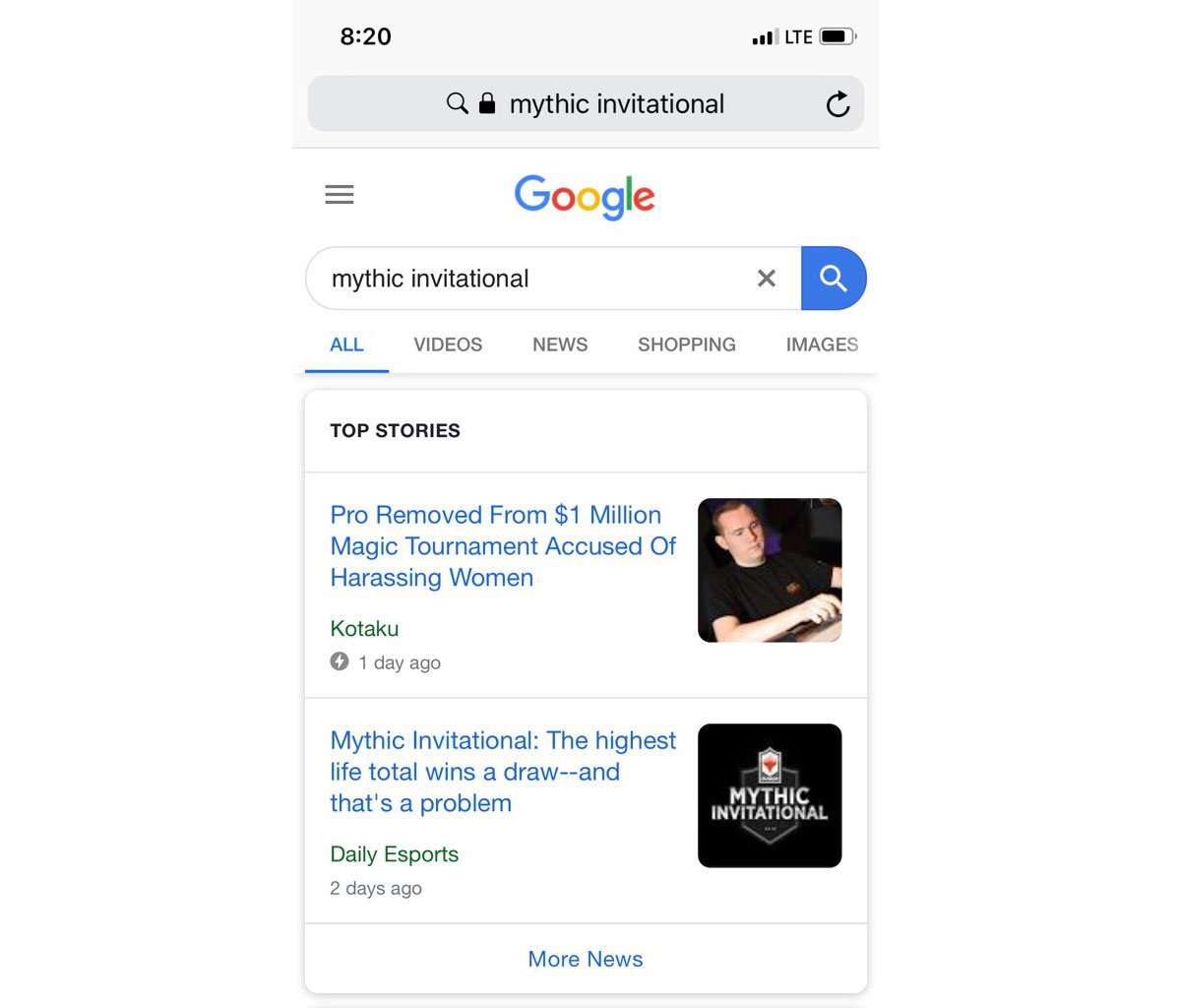This image portrays a mobile screenshot of a Google search result page taken at 8:20, as indicated by the black time display in the upper left corner. On the right side of the top bar, the signal strength icon shows four bars with three filled in black and the last one in gray, suggesting a strong signal. Next to the signal strength, the text LTE appears, followed by a horizontal battery icon indicating approximately 80% charge.

Beneath the time and signal indicators, the top of the mobile browser is visible. This section features a gray box with several icons: a magnifying glass, a black lock, and the text "Mythic Invitational". Towards the right of this box, there's a refresh icon. Directly below, the Google logo is prominently displayed on the left, adjacent to a three-horizontal-line menu icon.

The main body of the screenshot contains a text input box where the search query "Mythic Invitational" has been entered. At the far right of this box, there's an X icon for clearing the search text, with a blue button containing a white magnifying glass for initiating a search located externally to the right of the box.

Under this search input area, various tab options are displayed: All, Videos, News, Shopping, and Images. The 'All' tab is highlighted in blue, indicating it is the active selection.

The search results begin with the "Top Stories" section, marked by a black header and a thin gray line separator. The first news item in this section includes a square photo on the right of a man with a buzz cut wearing a black shirt. The accompanying headline, appearing in blue text to the left of the image, reads: "Pro Removed from $1,000,000 Magic Tournament Accused of Harassing Woman." Below this headline, the source name "Kotaku" is displayed in green, accompanied by a gray circle icon with a white lightning bolt inside and the text "One day ago" to its right. This news story is separated from the next by another thin gray line.

The following news result features an image on the right with a black square labeled "Mythical Invitational." The headline to the left states: "Mythic Invitational: the highest life total wins a draw – and that’s a problem" in blue text. The source, "Daily Esports," is listed in green beneath the headline, followed by "Two days ago" in gray text. Another thin gray line separates this item from additional content.

At the bottom of the visible content, centered in blue text, a link labeled "More News" invites viewers to explore further news stories.